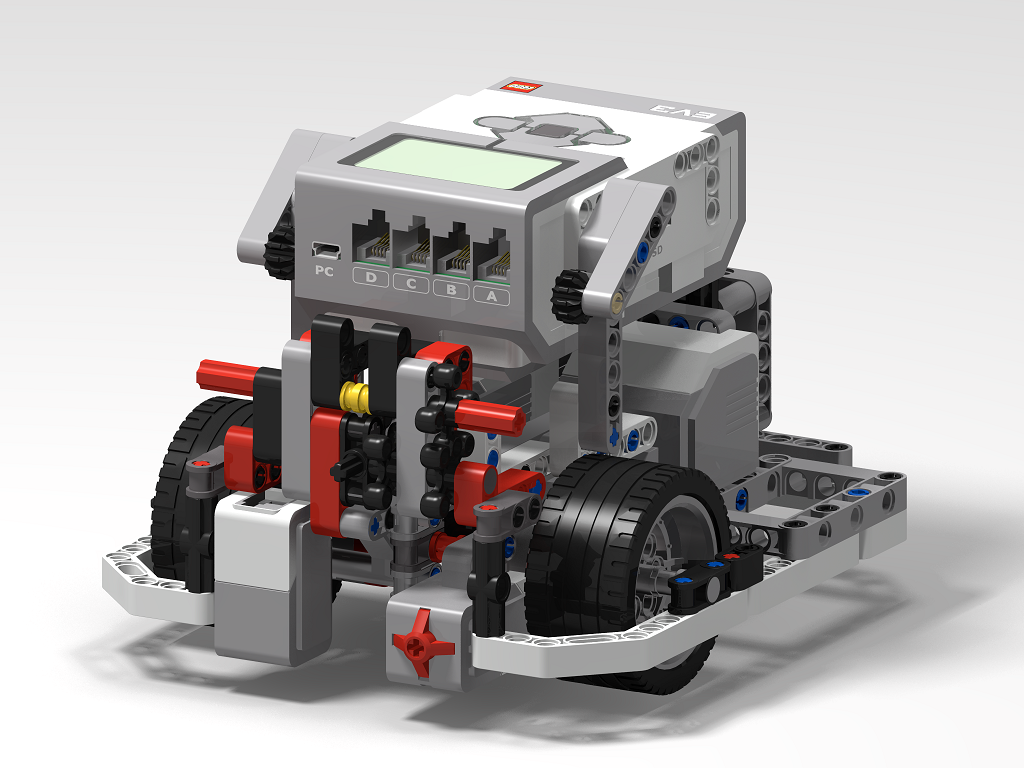In a brightly lit indoor setting with a predominantly white background, a meticulously assembled Lego creation is showcased. This intricate, machine-like model features a boxy, predominantly gray structure, accented with red and black pieces that suggest the presence of an engine. The creation is mounted on two wide, black tires positioned at the bottom left and right, giving it a sturdy and mobile appearance. 

At the top of the model, there are four clearly labeled ports marked PC, D, C, B, and A, resembling phone jacks where components could potentially be plugged in. These ports are aligned horizontally across the top face. Additionally, small red levers are visible on the front left and right sides, which might be designed to be pushed or spun. The machine is oriented slightly diagonally to the left, adding a dynamic element to its presentation. Shadows underneath the Lego creation provide depth and context to its three-dimensional form, while the background features subtle light blue hues, adding to the overall clean and detailed appearance of the image.